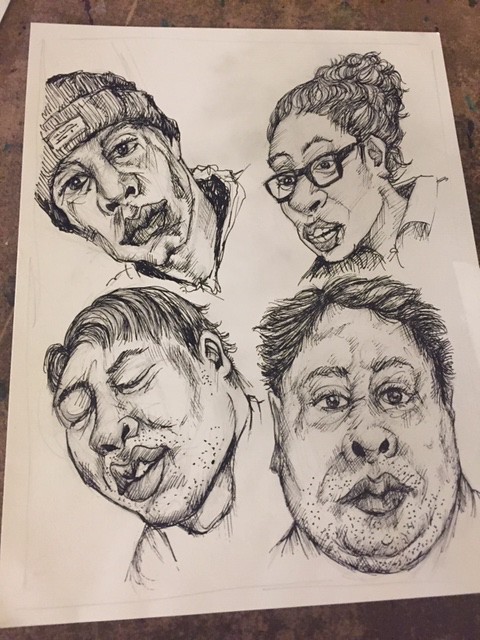On a cream-colored piece of paper placed on a brown stone surface, four detailed pencil drawings of faces are arranged in a two-by-two grid format. These illustrations, done in a caricature style with pronounced features and rich shading, present each individual's head and part of their shoulders. In the upper left, a black man wearing a brimmed wool cap with his head tilted slightly to the left; he has very large lips, a wide-featured nose, and partially shown hoodie top. To his right, the upper-right corner, is a woman with her hair pulled back in a bun, dark square glasses, and very large lips with her mouth slightly open to show her teeth. Her wide nose and the top of her shirt, resembling a college shirt, are also visible. In the bottom left corner, there is a man with short, dark, and straight hair tilting his head to the left, eyes closed, and a mouth with large lips slightly open. Lastly, in the bottom right, the largest head belongs to a man with short hair, eyes open, big lips, a less wide nose, and visible stubble around his chin, giving him a double chin. Each face distinct, yet unified by their exaggerated, expressive features and strong shading emphasizes the intricate detailing of the pencil drawings.